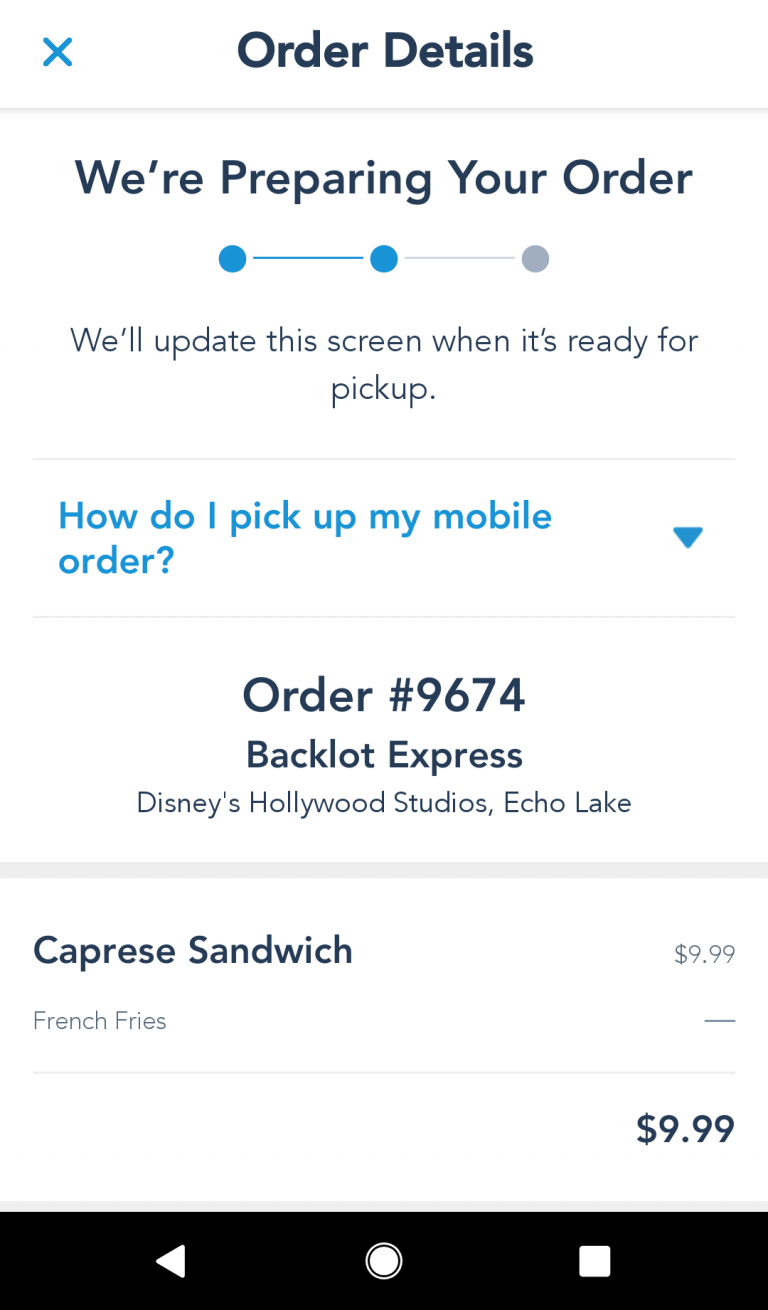The image depicts a mobile order confirmation screen for a pickup at Backlot Express in Disney's Hollywood Studios, Echo Lake. The screen has a vertical phone format, primarily with a blue and white color scheme. 

At the top of the screen, there is a blue header labeled "Order Details" with a blue "X" to the left of it, presumably for closing the window. Below this header, dark blue text states, "We're preparing your order," accompanied by a progress bar consisting of three dots connected by lines. The leftmost two dots are blue, indicating progress, while the rightmost dot is gray, indicating pending steps.

Underneath the progress bar, a message in standard font reads, "We'll update this screen when it's ready for pickup." Following this, there is a gray horizontal line. Beneath the line, a clickable option labeled "How do I pick up my mobile order?" is shown, indicated by a blue downward arrow.

Next, another gray line divides this section from the order details. In black text, the order number "Order Number 9674" is noted along with the location "Backlot Express, Disney's Hollywood Studios, Echo Lake."

Following the thicker gray divider line, the items ordered are listed. The first item, a "Caprici Sandwich," is in black text with a price of "$9.99" next to it. Below that, "French Fries" is indicated in smaller gray text without a specified price, also denoted by a gray line placeholder.

At the bottom right, in darker text, the total cost is reiterated as "$9.99." The bottom of the screen is occupied by a black bar featuring a white circle in the middle, with a left-pointing white arrow on the left side and a white square box on the right.